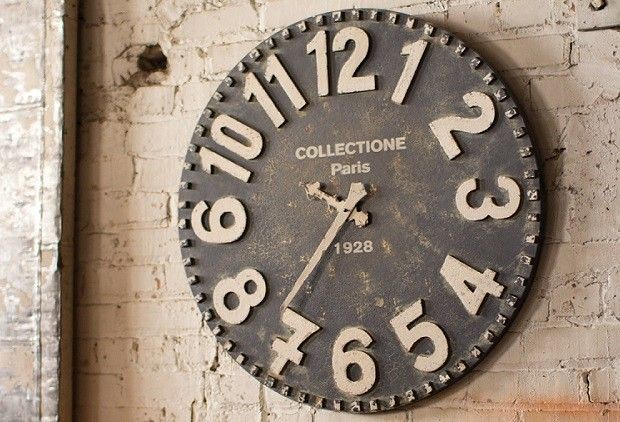A vintage clock, prominently featuring Roman numerals from I to XII, displays the time as 10:35 with the hour hand pointing towards 10 and the minute hand towards the 7th minute mark. The clock is part of an antique collection titled "Paris Collection" and has the year "1928" inscribed below its face. Surrounding the clock are various symbols etched into a backdrop of aged and cracked stone bricks, giving the scene a historic and weathered appearance. The left side prominently features a large, distinct stone brick, adding to the rustic ambiance of the setting.